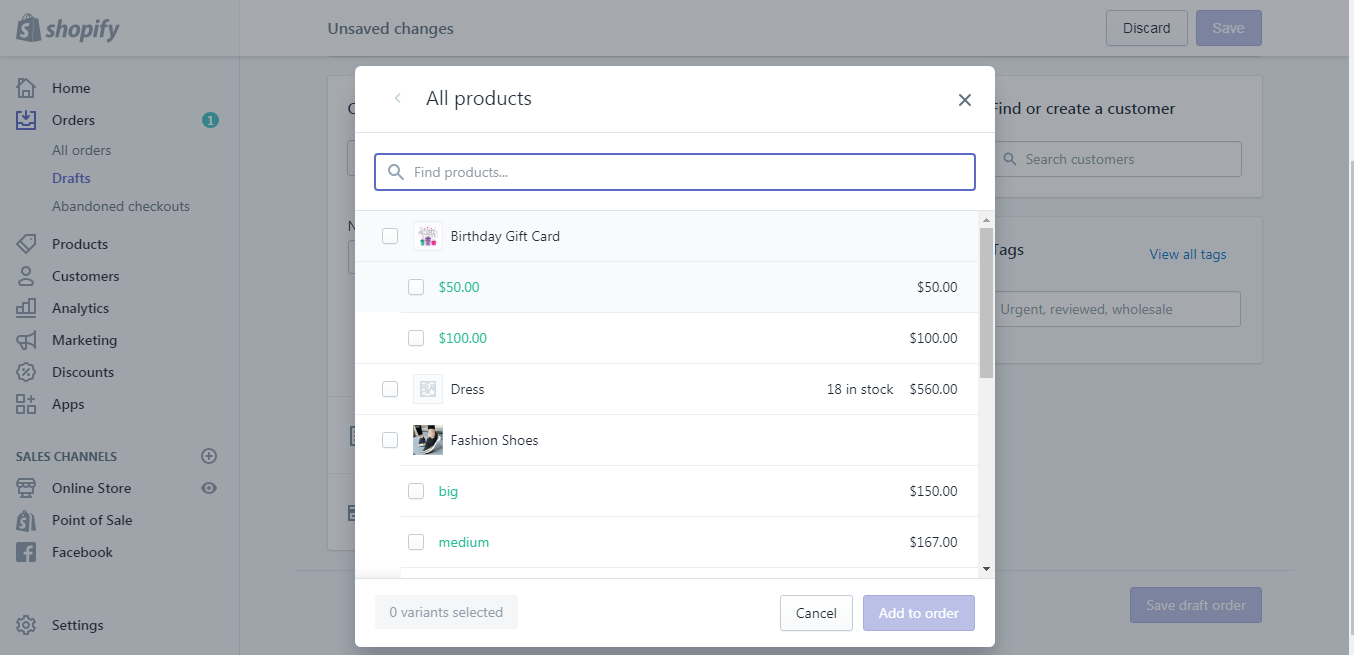A screenshot of the Shoplify dashboard is shown, featuring a clean and functional interface. On the left sidebar, menu options such as 'Home,' 'Orders,' 'Products,' 'Customers,' 'Analytics,' 'Marketing,' 'Discounts,' and 'Apps' are visible. These options are arranged vertically in plain text. Despite the simplicity and lack of flamboyant design, the layout appears intuitive, allowing easy navigation for users. 

An 'Orders' menu is expanded, offering more detailed actions. The focal point of the image is a pop-up dialog titled 'All Products,' which includes a search bar. Although no text has been entered into the search bar, several product listings are visible on the interface. The listings feature items such as "Birthday Gift Card" available in $50 or $100 denominations, a "Dress" with a stock quantity of 18, and various "Fashion Shoes" in different sizes, marked generically as Big and Medium. This generic labeling could indicate placeholders or simplified product descriptions within the broader context of a business inventory system.